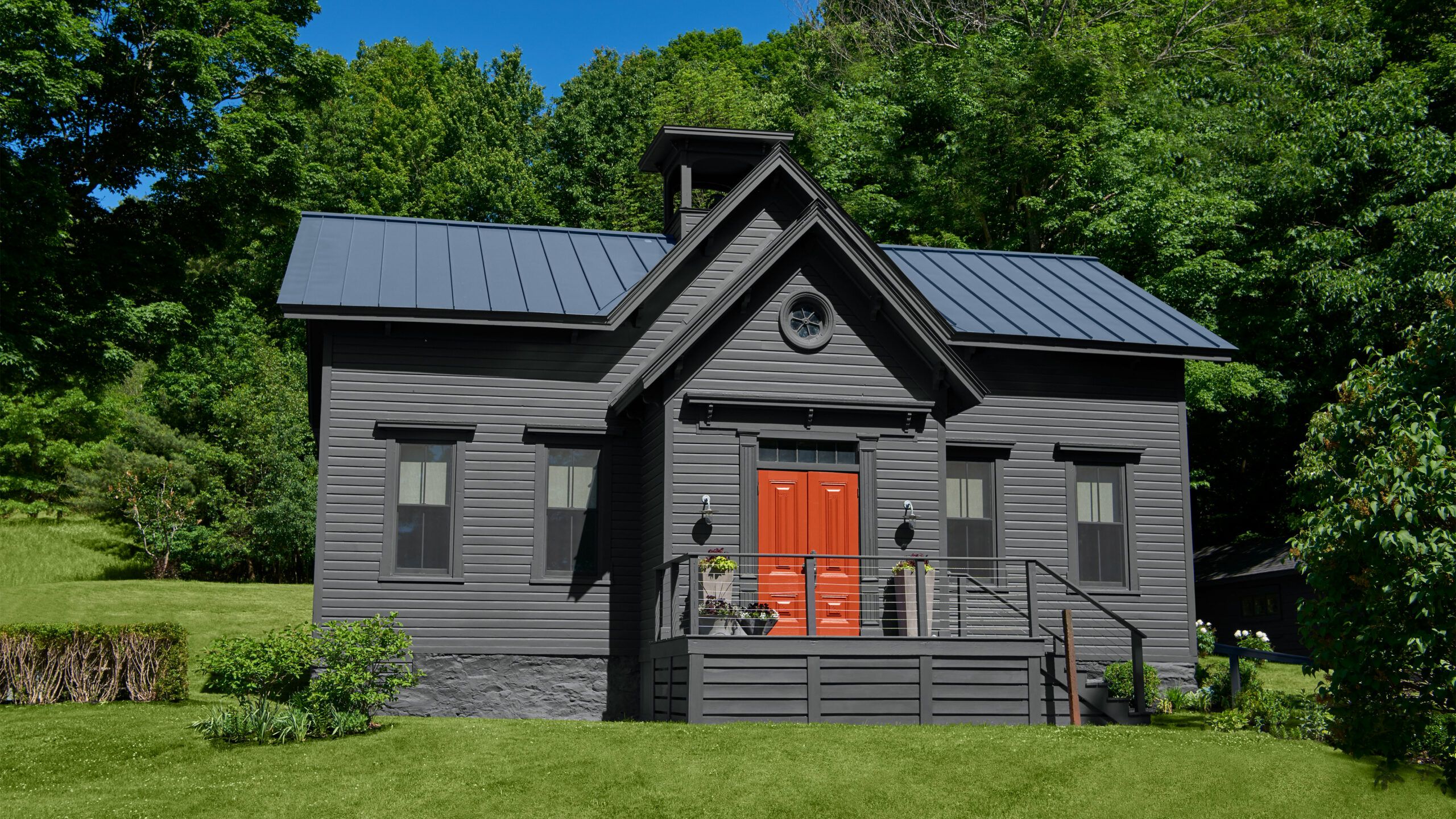This photograph captures a small, charming cottage nestled in a vibrant, green setting. The house is predominantly gray with an intriguing blend of architectural features, including a light blue, slatted roof that forms a triangular peak before leveling off, and a prominent chimney. The entrance is marked by a bright orange door, flanked by plant pots with greenery and dark purple leaves, as well as additional vases and plant arrangements. The front of the house is accessible via a staircase that leads to a quaint porch area. Surrounding the house are neatly trimmed green grass, bushes with green and brown branches, and a variety of flowers. The background showcases an array of leafy green trees under a vivid blue sky, with the sunlight illuminating the entire scene, adding to the vibrant and lively atmosphere of this picturesque setting.